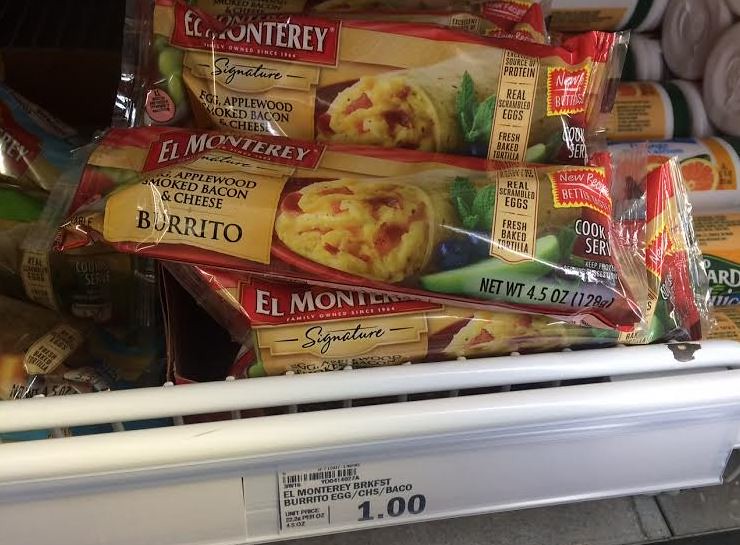The photograph showcases several packets of El Monterrey Breakfast Burritos neatly arranged on a supermarket shelf. Dominating the lower edge of the image is the white lip of the shelf, which prominently displays a price tag. The tag, detailing “El Monterrey Breakfast Burrito, Egg, Cheese, Bacon,” lists the price as $1 in large, bold black font. The burritos are packaged in long, rectangular red packages, adorned with the El Monterrey brand logo. Each package also features text stating "Egg, Applewood Smoked Bacon, and Cheese Burrito" along with a tempting image of the burrito, surrounded by colorful depictions of fresh vegetables.